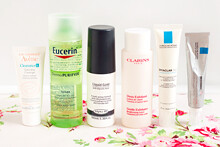A carefully arranged series of moisturizer and beauty products sit elegantly on a table adorned with a white tablecloth featuring a red floral design. The backdrop is a clean, minimalist white. From left to right, the array of products includes a triangular tube of moisturizer accented with pink and blue writing at the top. Following this, there is a transparent green cylindrical bottle of Eucerin, standing upright and catching the light. Next in line is a white cylindrical bottle with black writing and a prominent long black cap. This is followed by another white cylindrical tube, this time with red writing, adding a pop of color to the arrangement. Further along is yet another white cylindrical product, featuring black text and a distinctive turquoise square at the top. The final product stands vertically on its cap, showcasing a sleek design with a white cap, gray body, and a turquoise blue square near the top, completing the visually pleasing lineup.